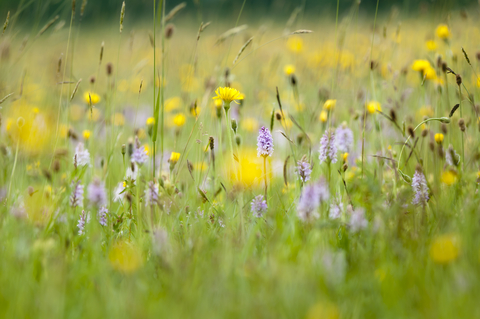The image captures a vibrant field of wildflowers and tall grasses under bright daylight. A close-up photograph, it showcases a rich array of flora with a mixture of light purple, pinkish, and yellow flowers across the scene. Prominently, clusters of fuzzy, lilac-colored flowers on long stems stand out amidst tall, wispy grass blades and patches of dandelions. Some grass stalks resemble tiny wheat heads, adding texture to the composition. Among these, small sunflowers with bright yellow petals provide a sunny contrast. The background fades into a blur of dark and light green shades mixed with more yellow and purple blooms, enhancing the depth and natural beauty of this outdoor wilderness snapshot. The overall impression is colorful and slightly overgrown, with a soothing blend of sharp and soft focus elements.